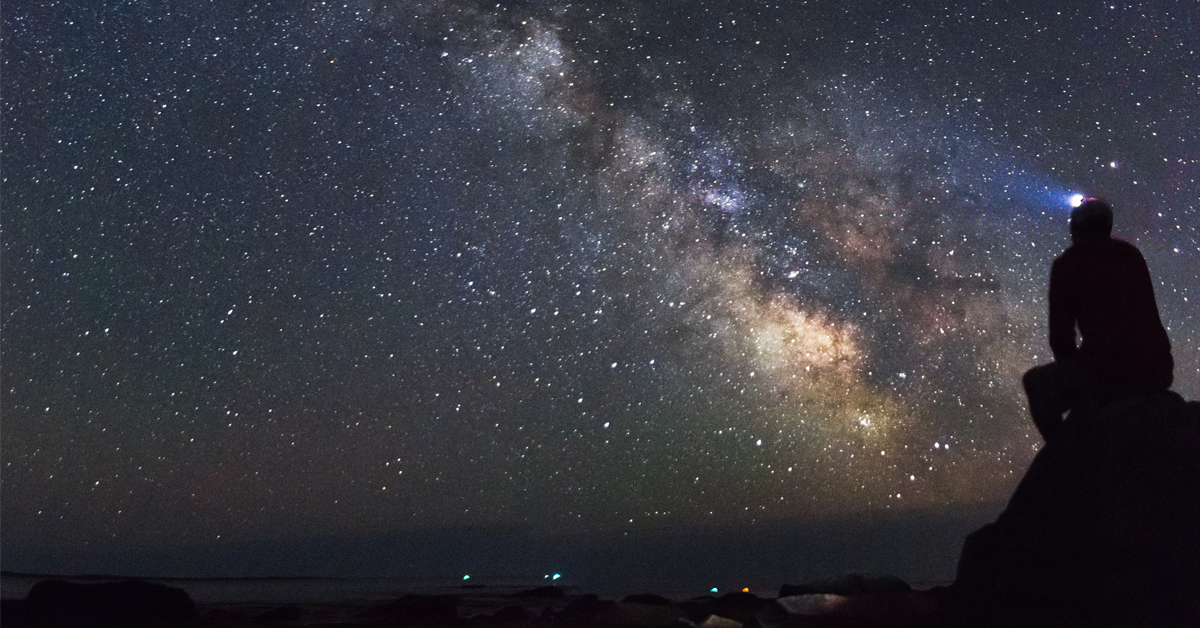The image captures a breathtaking night sky filled with countless stars, set against a deep, dark blue backdrop. A bright comet or cosmic ray cuts diagonally through the sky, adding an otherworldly glow. Below the vast celestial display, a lone figure, possibly a man, sits atop a mountain or large rock. He is equipped with a helmet that has a light attached, casting a small but noticeable glow around him. The person's silhouette is partially illuminated, contrasting with the immense, starlit expanse overhead. A faint outline of a town's lights twinkles at the base of the scene, enhancing the sense of scale and adventure. Overall, the image evokes a sense of awe and the wonder of exploring nature's night-time beauty.